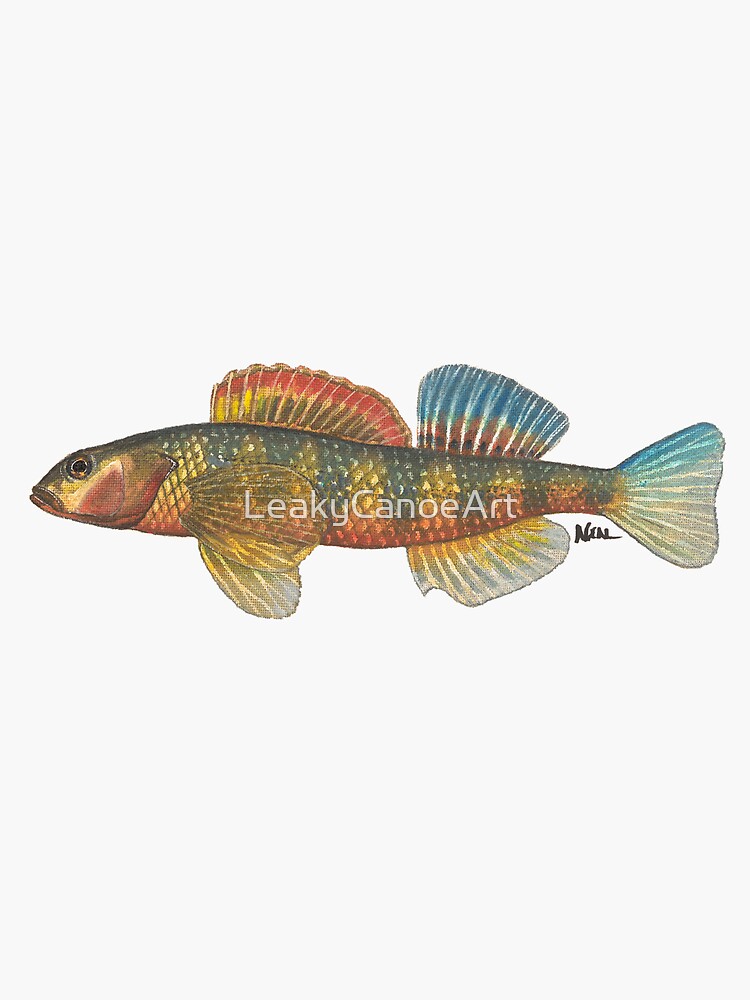This detailed illustration depicts an elongated fish positioned centrally against a white background, seemingly rendered on canvas as indicated by visible paint strokes and a faint canvas texture. The fish, exhibiting an array of bold, rainbow colors, showcases a head on the left and a tail on the right in a classic profile view. The spectrums of reds, yellows, greens, and blues are prominent across its scales, transitioning from a greenish-brown mouth area to a tan section under the eye, and further into a gold, red, and orange color scheme along its underbelly. The fish features two dorsal fins: the first fin is shorter and longer with a blend of red, gold, and brownish-green hues, while the second fin is distinctly blue. Additionally, the fish has two fins on its ventral side and a fin near the tail. The eye is gold with a black iris, and its mouth is closed. Near the tail, the artist's signature "Neil" is clearly visible in black paint, accompanied by the text overlay "Leaky Canoe Art." This image is displayed in a portrait layout, emphasizing its vertical elegance.